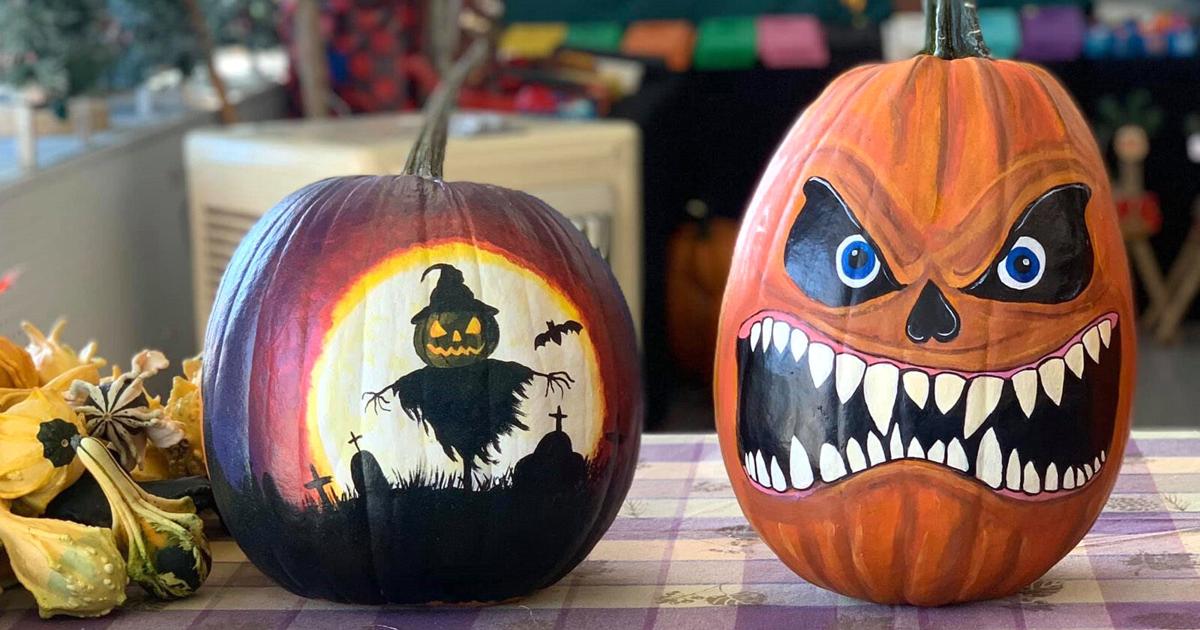This vibrant color photo showcases two exquisitely hand-painted pumpkins set on a purple and white checked tablecloth, surrounded by an assortment of small gourds. The background hints at an art studio, adding a creative ambiance with its out-of-focus splashes of pink, green, orange, and yellow.

The pumpkin on the left, round and painted in a purply-pink hue, features an intricate Halloween scene. It boasts a central image of a jack-o-lantern-headed witch flying against a large, yellow-rimmed moon. The witch, dressed in a black cap and scarf, sports a jagged scarecrow shirt with stick arms. Below her, a spooky graveyard with tombstones and silhouetted crosses stretches across the base. A bat flutters nearby, completing the eerie tableau.

To the right is a taller, more oblong pumpkin, striking with its ominous features. Painted in vibrant orange, it displays menacing black eyes with a hint of blue, an upside-down heart-shaped nose, and a wide, snarling mouth brimming with razor-sharp teeth extending to the sides. This stark contrast in artistic styles between the pumpkins highlights their Halloween-themed decorations, making them a perfect centerpiece for the season.